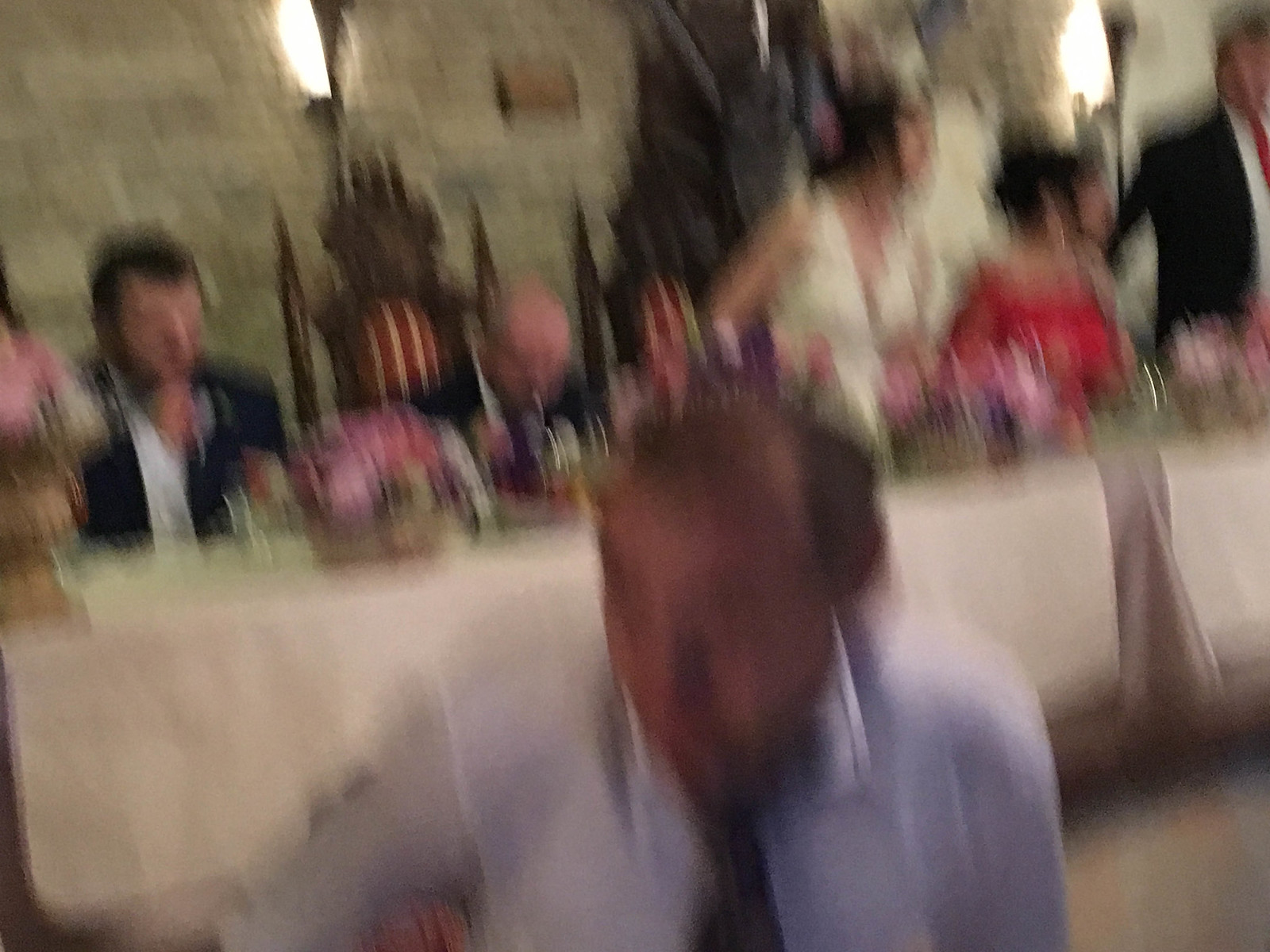The image is an extremely blurry photograph, likely taken during a wedding reception. It captures a long, white table spanning from left to right, adorned with magenta and pink flowers. Seated at this table are several people: starting from the left, there are two men—one in a blue suit with a pink flower on his shoulder, and another bald man, possibly wearing a dark-colored suit, caught mid-drink. Beside them, a woman in a white dress, possibly the bride, with black hair and wearing a tiara, is either seated or in the motion of standing up. Next to her is a woman in a red dress with black hair and glinting earrings. Further to the right, another man in a black suit with a white shirt and a red tie is partially visible. Centered in the foreground, closer to the camera, is a man with a receding hairline, wearing a white shirt and a dark-colored necktie, looking towards the left bottom section of the photo. The backdrop features high-backed, striped, throne-like chairs against a wall with two light fixtures, enhancing the regal ambiance of the scene.